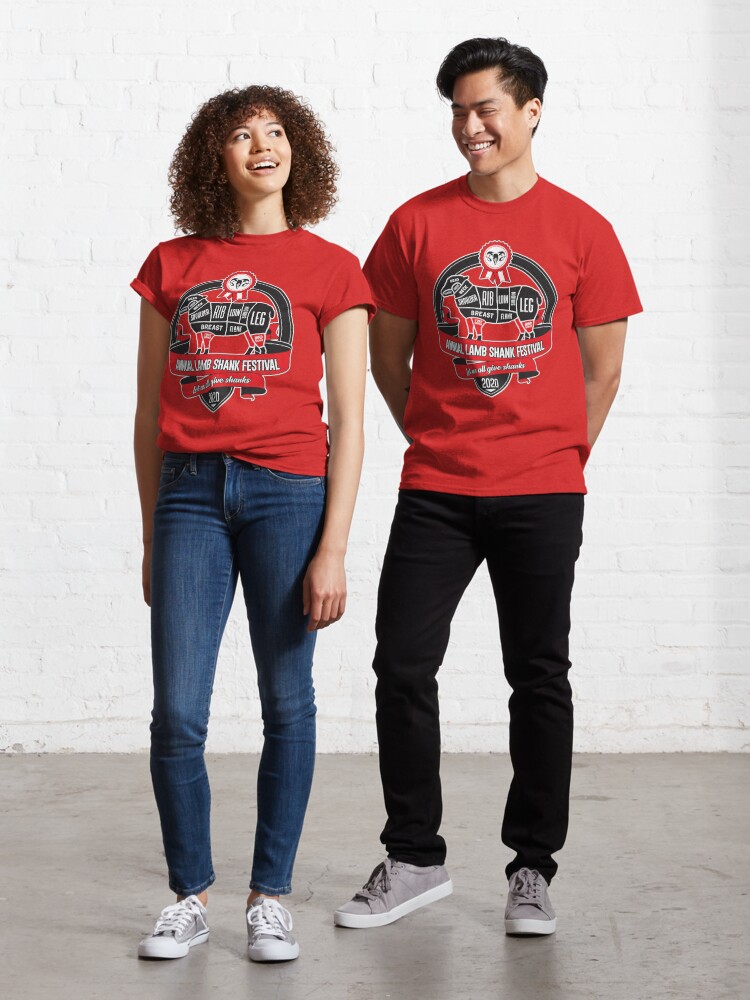In this vibrant photograph, two young people, likely in their 20s, are standing joyfully in front of a white brick wall on a gray concrete floor. Both are dressed in matching red T-shirts emblazoned with "Annual Lamb Shank Festival" in white text, accompanied by a detailed illustration of a black sheep. The sheep is segmented to show different cuts such as the leg, shank, brisket, and rib, with blue markings.

The girl, positioned on the left, has dark brown, shoulder-length curly hair, and is looking up with a smile. She wears light blue jeans and gray tennis shoes with white laces, with her toes pointed towards the camera and her arms hanging at her sides.

The boy, standing to her right, appears to be of Asian descent with short black hair. He is smiling as he looks slightly down towards her. He is dressed in darker jeans and similar gray tennis shoes. His right leg is bent with the heel off the ground, and his hands are held behind his back. Together, they create a warm and inviting image, showcasing their happy spirits and shared enthusiasm for the festival.